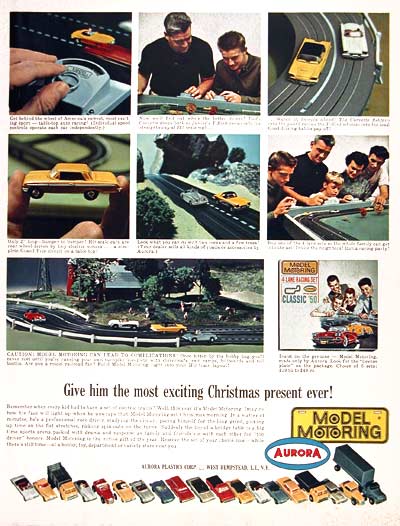The image is a digital screenshot of an advertisement for Model Motoring by Aurora, promoting it as "the most exciting Christmas present ever." The ad features several colorful pictures showcasing the toy model cars and track. Central to the ad are images of the yellow, white, blue, and red model cars racing on a large, electric track. This detailed track is set against a backdrop of a farmhouse, trees, and people on the grass, enhancing the scene's realism. Across different blocks of the ad, we see people engaged with the product: one image shows one or two men admiring the white car, and another depicts a group of men and boys gathered around the racetrack. Additional photos include a close-up of someone holding a model car and two individuals playing with the cars. The overall composition effectively combines vivid visuals and engaging content to draw attention to the toy's excitement and appeal.